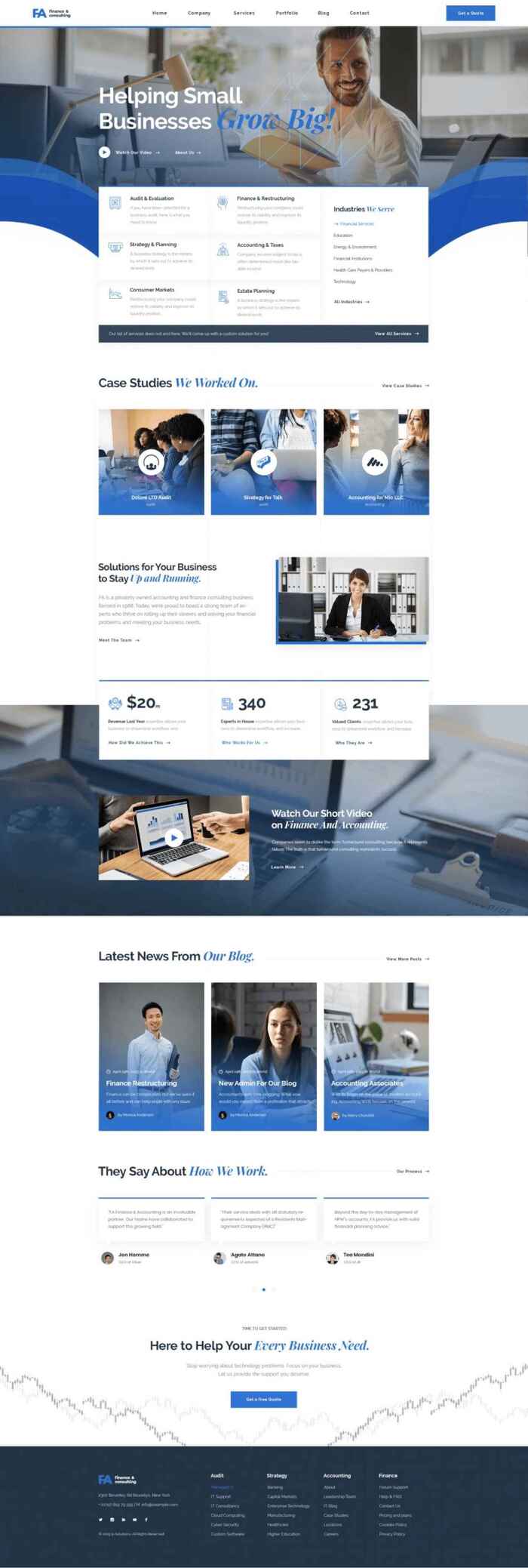In the photographic image, we see a zoomed-out view of a web page dedicated to promoting services that help small businesses grow. Dominating the page is a header with the tagline "Helping Small Businesses Grow," accompanied by a smiling man. The phrase "Grow Big!" is prominently displayed in blue, along with an exclamation mark for emphasis.

At the center of the web page is a white panel filled with various numbers, which are difficult to decipher due to the small font size. Surrounding this panel are vibrant hues of blue, white, and dark blue, creating a dynamic visual experience.

The page features images of people, including a woman sitting at a desk who appears to embody the professionalism of corporate America. Specific numbers such as "20," "340," and "231" are scattered throughout the content, although their exact significance is unclear.

Towards the bottom of the page, there is what seems to be an advertisement for internet services. It showcases workers engaged in different activities — a man in a button-down shirt is holding a tablet, and a girl is in conversation, reflecting a collaborative work environment. Additionally, an open laptop is visible, displaying sections like "They Say About How We Work" and "Latest News From Our Blog," hinting at positive testimonials and recent updates.